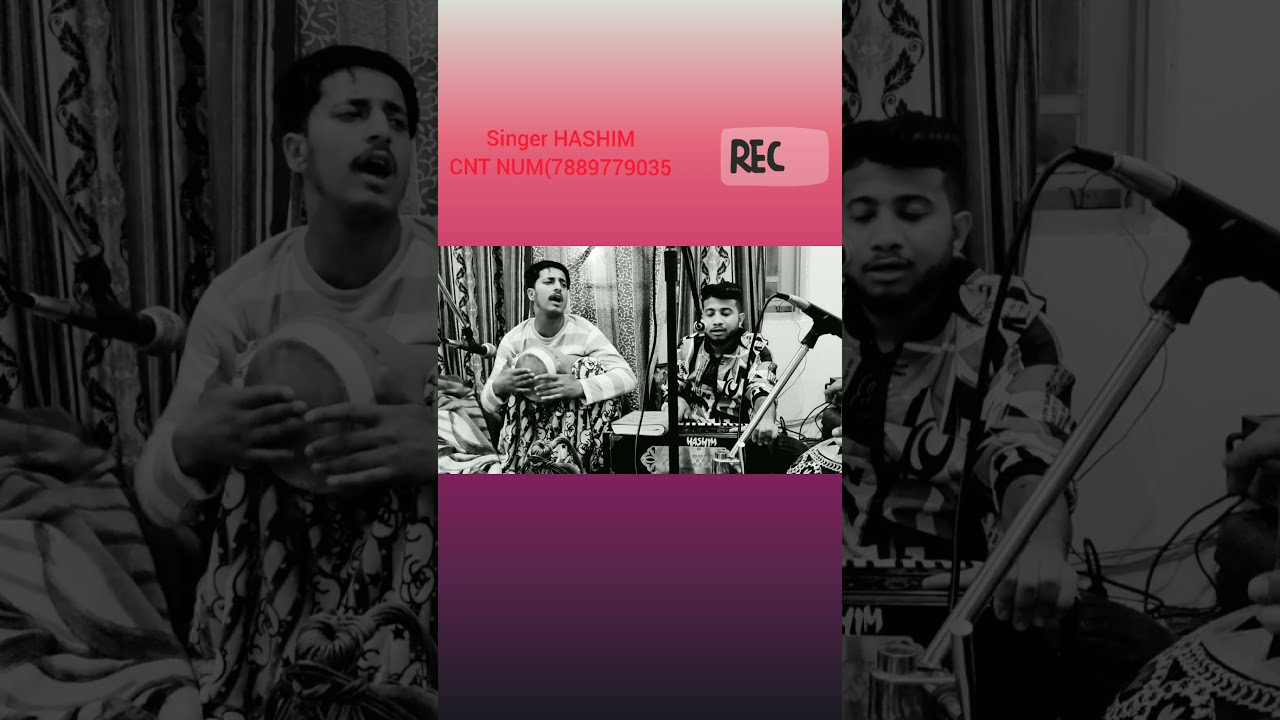This image features a vertically oriented poster with a gradient background transitioning from white at the top through pink to a deep purple at the bottom. Central to the image is a smaller black-and-white photograph placed over an enlarged version of the same photo, creating a layered effect. The photo captures two men, possibly of Middle Eastern descent, engaged in a musical performance. 

The man on the left is depicted playing a hand drum with his eyes open, while the other, on the right, appears focused on a keyboard with eyes closed. Both men are singing into microphones. Above the photo, a pink header contains the text "Singer Hashim" in darker pink, followed by the letters "C-N-T-N-U-M" and a phone number, "788-977-9035". Directly underneath this, there's a small, light pink button labeled "REC" in black text, likely indicating a recording button. The footer of the smaller photo is purple, enhancing the ombre effect of the background. 

Decorative elements such as brightly patterned curtains and possibly a blanket held by the man with the drum can also be seen in the photo, though they remain in black-and-white. The entire composition effectively combines detailed textual information with a poignant musical scene, accentuated by the gradient color scheme.